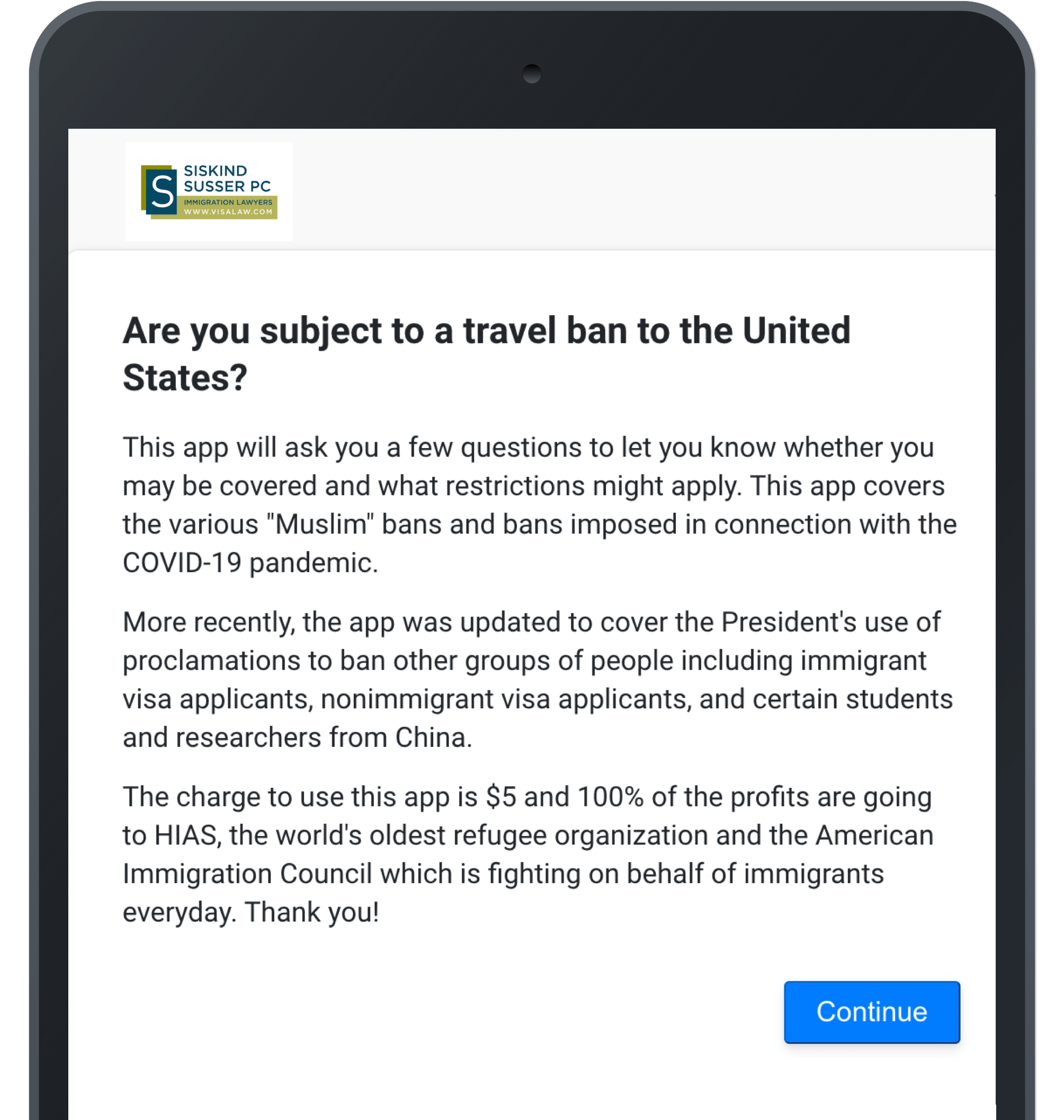This image, sourced from a website, is set against a white backdrop and framed by a black outline. In the top left corner, there is a forest green square containing a white "S." Behind it, there is a larger sage green square. To the right, the text "CISKIND" is displayed in sage green, followed by "SUSSER" and the letters "PC." Beneath this, a sage green box with green text at the top and white text at the bottom is present, though the content is illegible. A thin gray line separates this section from the subsequent content below.

In bold black text, the question "Are you subject to a travel ban to the United States?" is posed. Below, a paragraph states: "This app will ask you a few questions to let you know whether you may be covered and what restrictions might apply. This app covers the various 'Muslim' bans and bans imposed in connection with the COVID-19 pandemic." 

The following paragraph reads: "More recently, the app was updated to cover the president's use of proclamations to ban other groups of people, including immigrants, visa applicants, non-immigrant visa applicants, and certain students and researchers from China."

Continuing, it mentions: "The charge to use the app is $5, with 100% of the profits going to HIAS, the world's oldest refugee organization, and the American Immigration Council, which is fighting on behalf of immigrants every day."

The section concludes with a "Thank you!" followed by a blue box in the bottom right corner that reads "Continue" in white lettering.